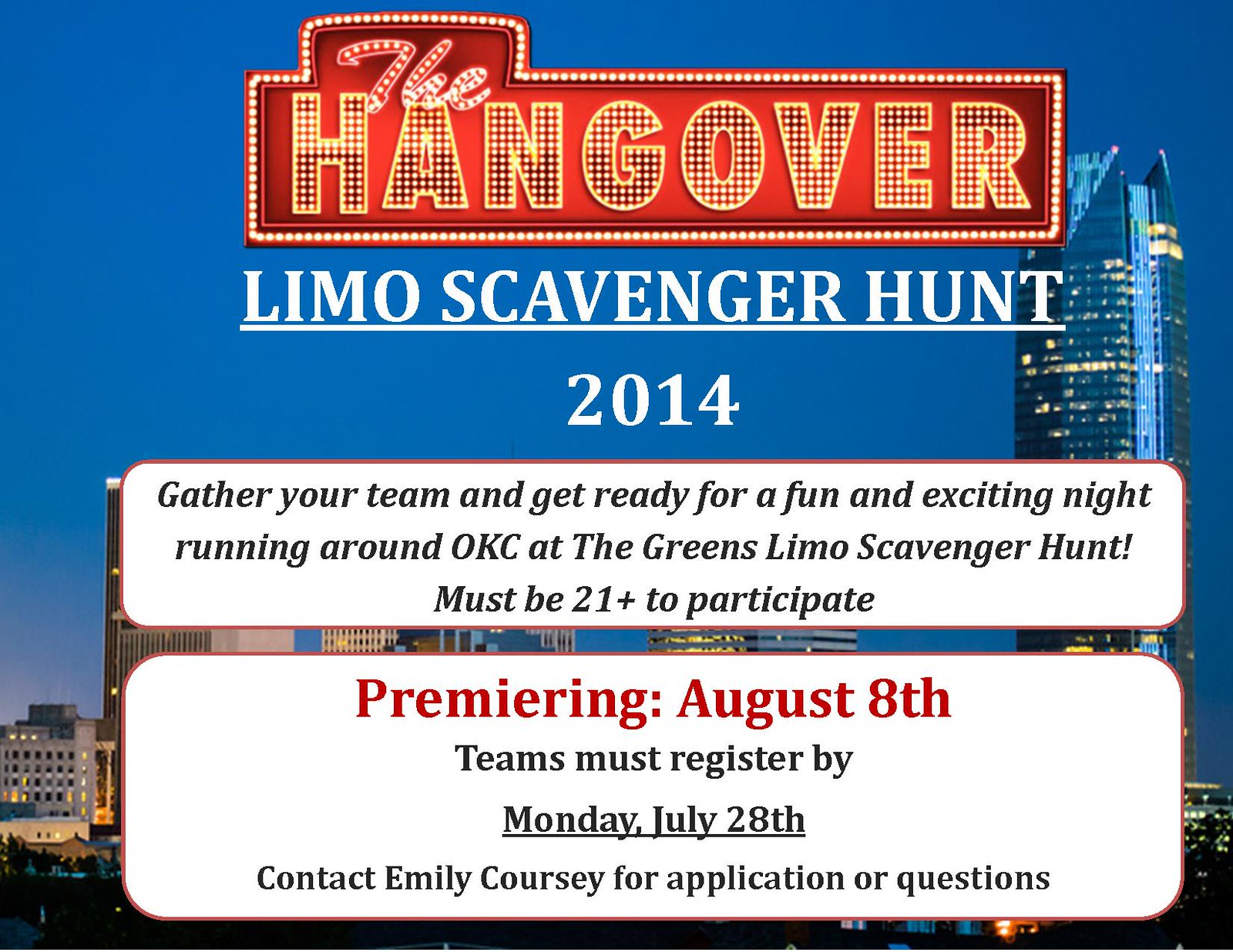The image is a promotional collage showcasing an event set against a city skyline, possibly Oklahoma City, at dawn or dusk. The background features a vibrant royal blue sky with an array of buildings, some six stories high and others towering up to 50 stories with shiny metal façades.

Overlaying this cityscape, the focal point is a banner resembling a neon nightclub sign that reads "The Hangover" in illuminated, yellow dotted text, bordered by light. Directly below, in bold, white, underlined text, it states "Limo Scavenger Hunt" followed by "2014." Beneath this, a white text box with black writing heralds the event details: "Gather your team and get ready for a fun and exciting night running around OKC at the Greens Limo Scavenger Hunt. Must be 21 plus to participate." 

At the bottom, an additional white text box with a red border announces: "Premiering August 8th" in red font, followed by further instructions in black text: "Teams must register by Monday, July 28th. Contact Emily Coursey for application or questions." This comprehensive and detailed announcement invites participants to join a thrilling scavenger hunt adventure throughout the vibrant city of Oklahoma City.